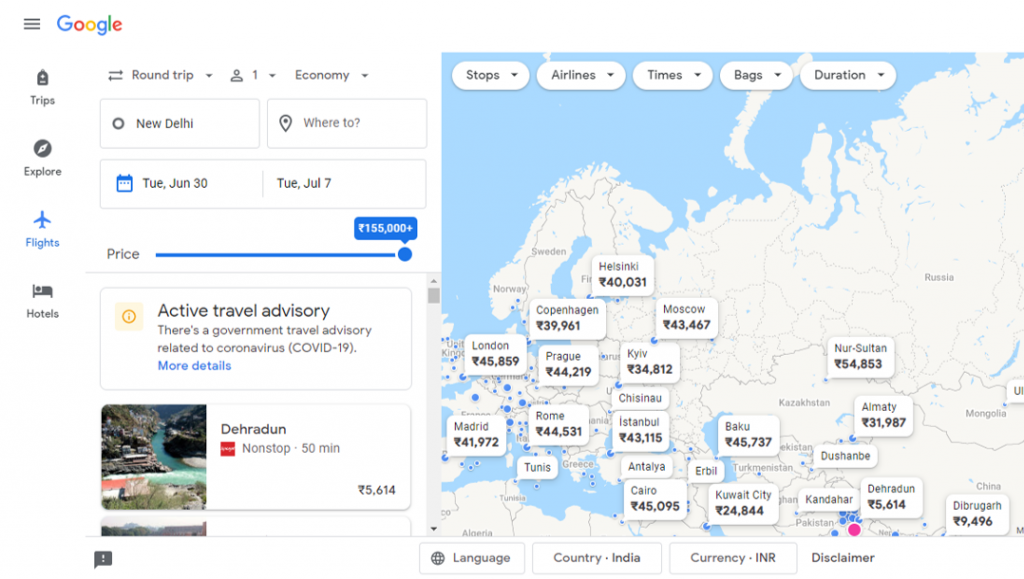The image is a detailed interface of Google Travel, prominently displaying various options for booking trips, flights, and hotels. In the upper left corner, the Google logo is visible, followed by a vertical menu on the left side featuring the options: Trips, Explore, Flights (highlighted in turquoise), and Hotels, all in black font.

To the right, there is a booking summary indicating a round trip with a left and right arrow icon below it. A small person icon with the number "1" next to it signifies one traveler, and the word "Economy" is accompanied by a down arrow for further options.

The main interface features horizontal rectangular input fields with black font on white backgrounds. The first field reads "New Delhi," while the second field is labeled "Where to." Below these fields is a turquoise calendar icon, with dates specified as "Tuesday, June 30th" on the left and "Tuesday, July 7th" on the right. Below the calendar details, there is a price slider represented by a turquoise line ending in a circle, with the value "155,000+" above it (the currency is unclear).

An active travel advisory is prominently displayed, stating government travel advisories related to coronavirus (COVID-19), with a turquoise link labeled "More details." 

Further down, the interface shows "Dehradun" spelled out, followed by a small red rectangle indicating a "Nonstop" flight duration of 50 minutes. An image representing Dehradun is aligned to the left of this information.

On the right side of the interface, there is a map, and at the top, you can see various categories with pull-down menus. These are arranged from left to right and include Stops, Airlines, Times, Bags, and Duration, all in black font within horizontal white oval areas.

Below these categories, several cities, each in its horizontal rectangular block, are listed. For instance, Copenhagen, Moscow, Cairo, Madrid, and Rome, each with respective prices displayed underneath.